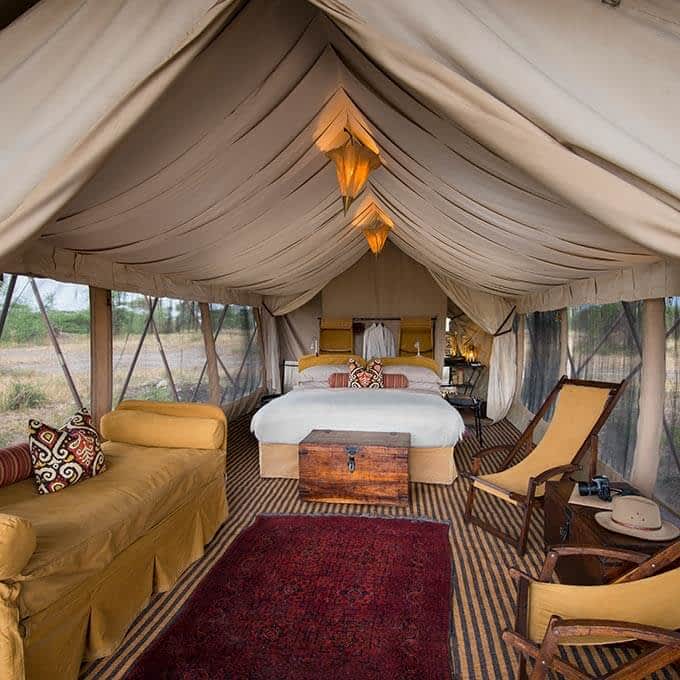This photograph showcases a spacious and luxurious tent that serves as an outdoor bedroom. The tent, adorned with a large, flowing cream-colored canopy that billows to a peak in the center, features high ceilings and hanging lights for illumination. The walls are lined with mosquito netting windows, offering views of a grassland with scattered trees beyond.

Inside, a white bed rests on a wooden frame at the center, flanked by various pieces of furniture. In front of the bed is a sizable, dark brown wooden chest, and a richly colored red and purple rug spreads out beneath. To the left stands a yellow couch adorned with a patterned white and orange pillow, set on a light and dark brown striped floor. To the right, a wooden table displays a hat, and two yellow cushioned chairs with dark brown frames complete the setting. This detailed and inviting setup highlights the blend of comfort and elegance within the expansive tent.